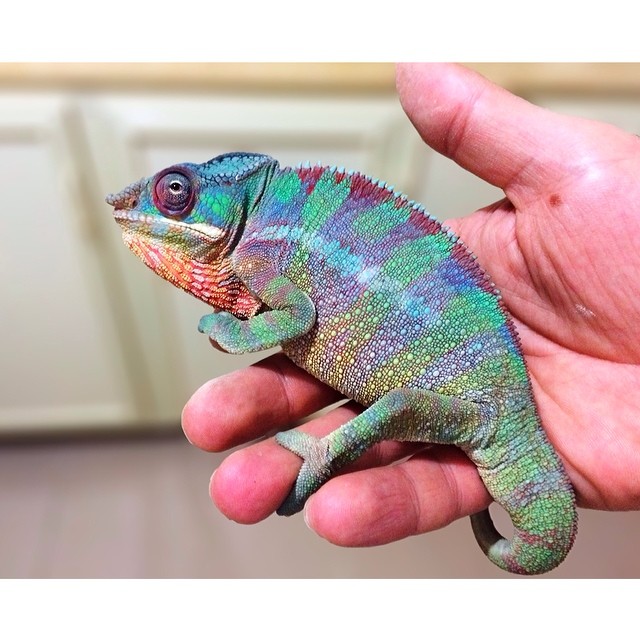In this photograph, a vibrant chameleon rests in the palm of a person's right hand, which belongs to a white individual. The chameleon is held with its head facing left and its tail slightly curved towards the bottom right. It clings to the person's finger with its back feet while its front legs are tucked beneath its head. This colorful lizard displays an array of pastel hues: a soft purple, green, and a striking wine red along its back, interspersed with blue vertical stripes. A splash of yellow and orange highlights its throat area, adding to its stunning appearance. Its eyes, exhibiting a pinkish-blue hue, are open and observant, while its small gray nose and closed mouth contribute to its serene expression. The chameleon's head is adorned with shapes resembling rabbit ears, though they are connected rather than free-standing. In the blurred background, white cabinets and a tan shelf are discernible, suggesting an indoor, possibly kitchen setting.